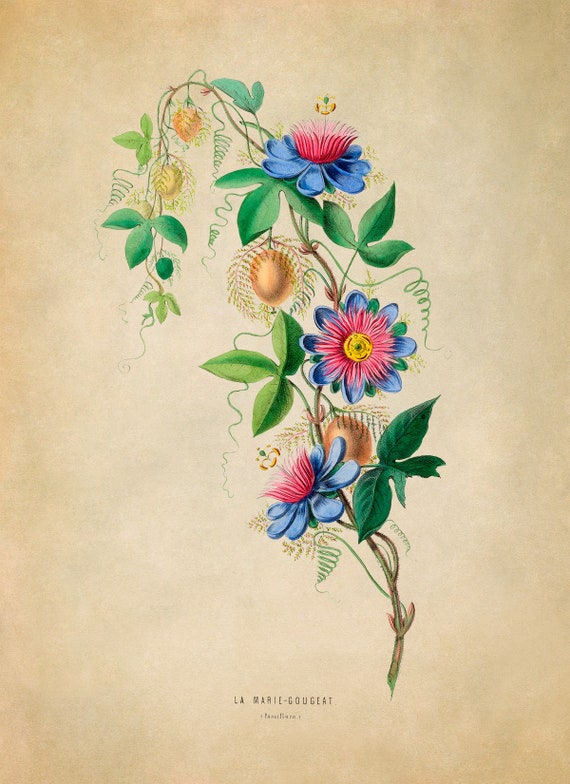This detailed artwork is a hand-drawn piece on a vintage-looking, mottled background of light and dark brown tones, displayed in a rectangular, portrait orientation. At the bottom of the drawing, French text identifies the piece, potentially including the name "L. Marie-Goudgeat" and a word resembling "Perifloral," written in dark font. The central focus of the drawing is a plant with a brown and green stem that extends diagonally from the bottom right to the top left of the page. This stem bears multiple green leaves arranged in threesome clusters along its length.

Three distinct flowers blossom from this plant, each featuring a harmonious blend of colors. The outer petals are blue, transitioning to reddish-pink petals towards the center, and culminating in bright yellow petals at the very heart of the flowers. In addition to these vibrant blooms, there are four closed flower buds in hues of yellow and orange, resembling small golden bulbs. These elements collectively create a rich tapestry of botanical life, juxtaposed against the earthy background, capturing a timeless and intricate depiction of nature.